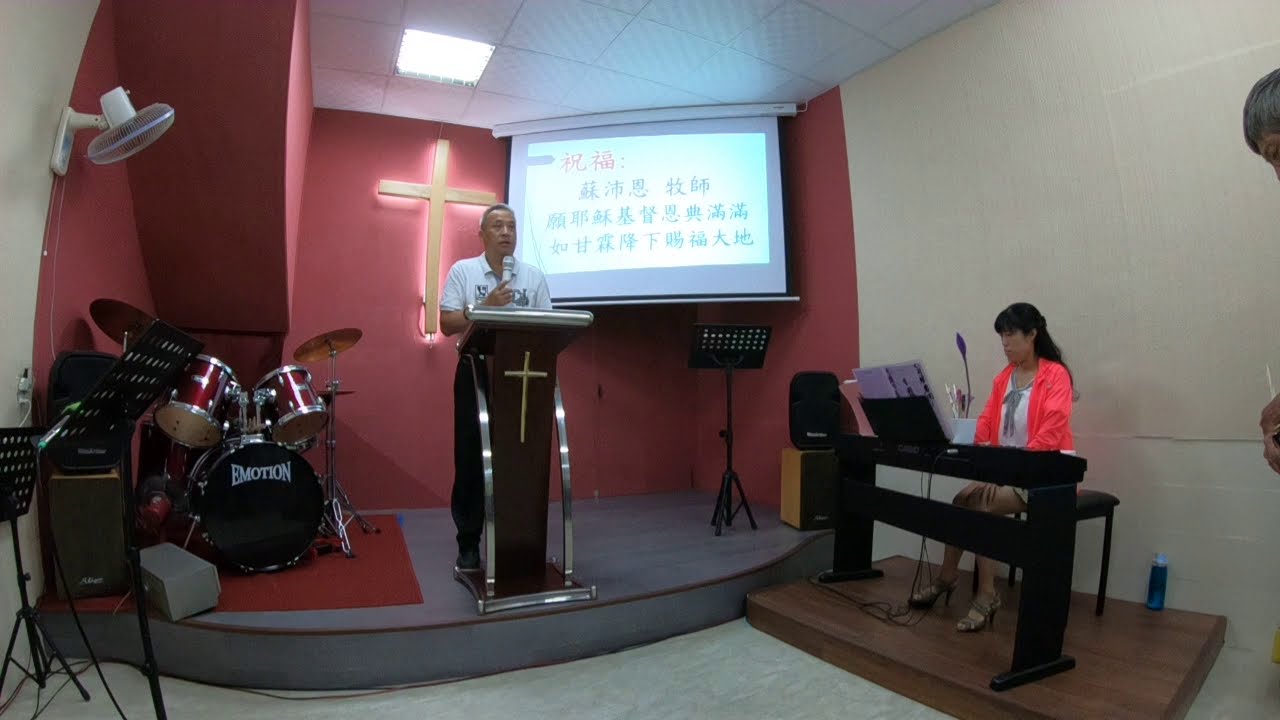The image depicts a church scene, possibly in East Asia, characterized by its identifiable interior and participants. Centered on a raised chancel area, a man dressed in a white polo shirt and black pants stands at a narrow wooden podium adorned with a gold cross, holding a microphone. Behind him, a large illuminated cross is prominently displayed on a dark red wall. To his immediate right, a projector screen with likely Korean or East Asian script is visible. In front of the screen, a woman with dark hair, wearing a bright orange jacket over a white top and a skirt, is seated at a black keyboard stand, with sheet music propped up in front of her. This section is demarcated by eggshell white walls. Further to the left on the dais is a drum set labeled “Emotion,” positioned beneath a fan mounted on the wall. The drum set is unoccupied. Additional music stands can be seen near the base of the dais, contributing to the structured yet intimate atmosphere of the gathering.